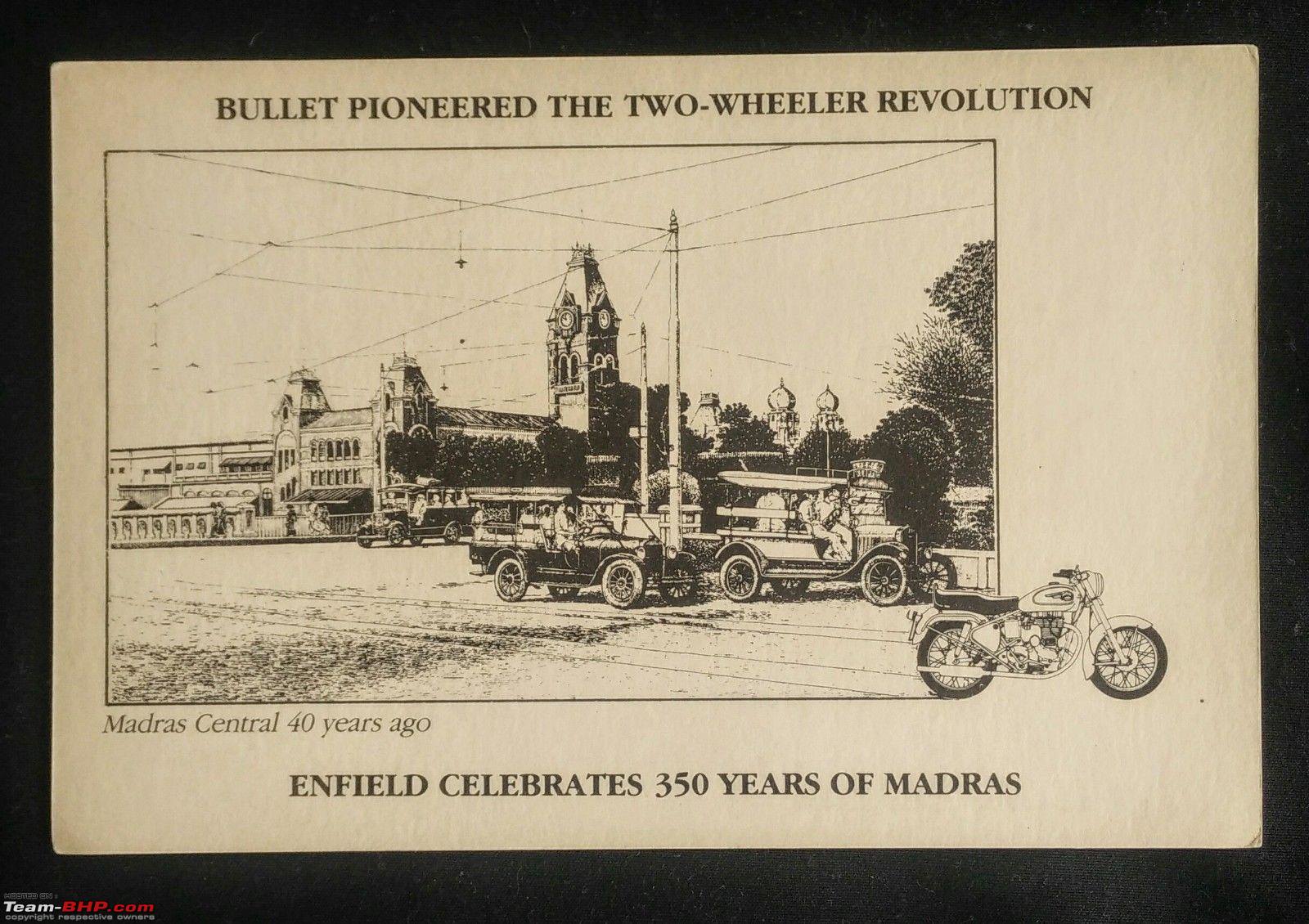This image portrays a poster or card that delves into historical themes, primarily featuring a hand-drawn, black-and-white cityscape. The central drawing captures a nostalgic street scene populated with early 20th-century vehicles, potentially dating back to the 1910s, including notable details such as a motorcycle illustrated on the right side, which slightly protrudes outside the main rectangular frame. The background showcases an old building crowned with a clock tower.

A network of wires, seemingly a grid formation, is seen hovering above the street, anchored by poles. Surrounding the street, trees add depth to the urban landscape. Dominating the top of the image, bold, capitalized text heralds, "BULLET PIONEERED THE TWO-WHEELER REVOLUTION." Below the artistic depiction, in smaller letters, it states, "Madras Central 40 years ago." Further down, in larger black letters, it proclaims, "Enfield celebrates 350 years of Madras."

The entire artwork sits against a cream background and is encased by a black border. A website, "team-bhp.com," is discreetly noted in the bottom left corner of this border.